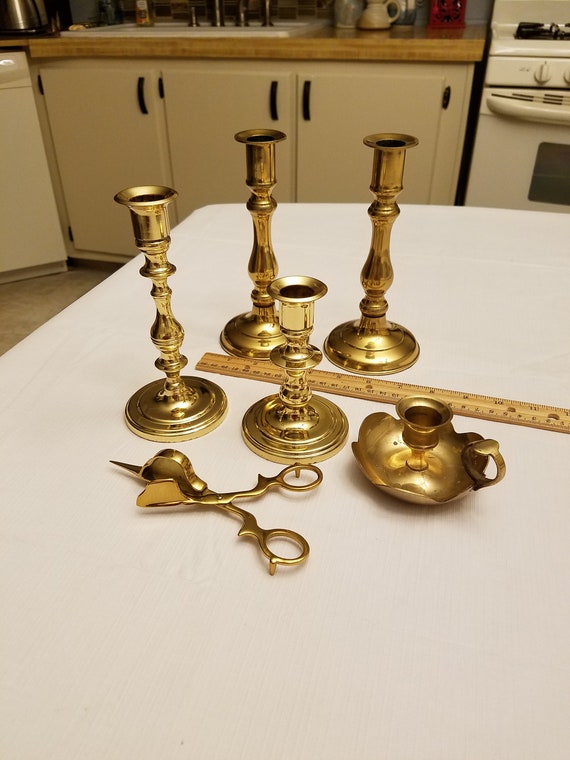The image depicts a detailed kitchen scene featuring a white tabletop adorned with various gold-plated candle holders and utensils. Central to the composition are four tall, shiny candlesticks with round bases, arranged in a square pattern; three are of identical height while the fourth is shorter. To the right of these candlesticks is a distinctive bowl-shaped candle holder with a handle. Nearby, a scissor-like wick cutter rests on the tabletop, and a brown wooden ruler is placed horizontally for scale. The background showcases white kitchen cabinets with black pulls, a butcher block countertop, a white gas stove with visible burners and knobs to the right, and a dishwasher to the left. The table, possibly covered with a large tablecloth, enhances the focal gold objects set against the light brown wood and white surroundings.